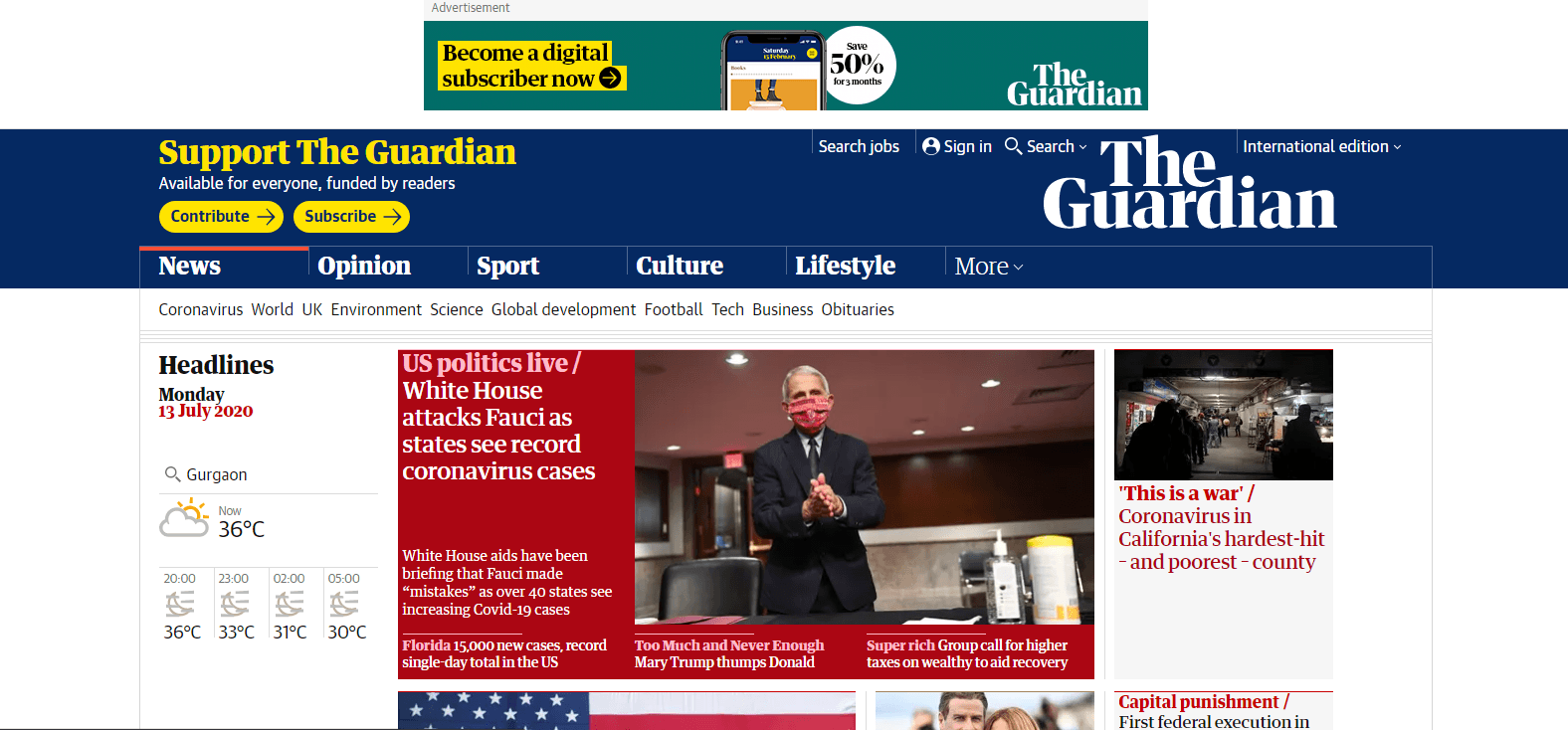The image displays a digital advertisement for The Guardian newspaper. At the top, there is a turquoise rectangle with a promotional message. Inside a yellow triangle, the text reads, "Become a digital subscriber now." Below this triangle, there is a depiction of a mobile phone and a circular graphic indicating a 50% discount offer. The primary branding text, "The Guardian," is prominently featured.

As you scroll down, the message, "Support The Guardian," appears, followed by the phrases "Available for everyone," "Funded by readers," and "Contribute or subscribe." There are also navigational options such as "Search jobs," "Sign in," and "Search The Guardian International Edition."

The website is divided into various sections: News, Opinion, Sports, Culture, Lifestyle, and more. Headlining the page is the date "Monday, 13 July 2020" written in red. The current weather, marked at 36 degrees, is displayed, with additional details for different times of the day.

The main content highlights a news blog titled "U.S. Politics Live," discussing recent attacks by the White House on foreign states and an escalation in record coronavirus cases.